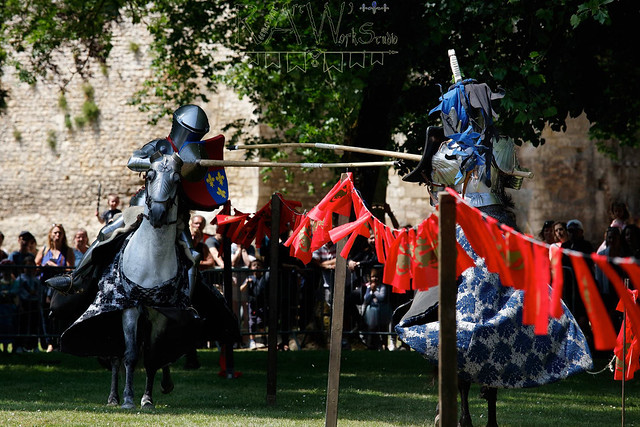This detailed photograph captures a lively jousting demonstration at what appears to be a Renaissance or medieval fair. In the foreground, two knights on horseback are poised for action, each clad in full metal armor and holding long, wooden jousting lances. The knight on the left is adorned in a black and white cloak with his horse's nose also protected by armor, while the knight on the right wears a blue and white cloak and a uniquely designed square helmet with a white extension. Both knights hold shields and aim their lances towards each other, separated by a wooden fence draped with orange-red banners. They are stationed on a grassy field, not yet in motion. The scene is set against the backdrop of a large brick building that resembles a castle, with many spectators gathered behind the fence to watch the spectacle. Additionally, there are trees framing the upper corners of the image, completing the historical ambiance of the event.